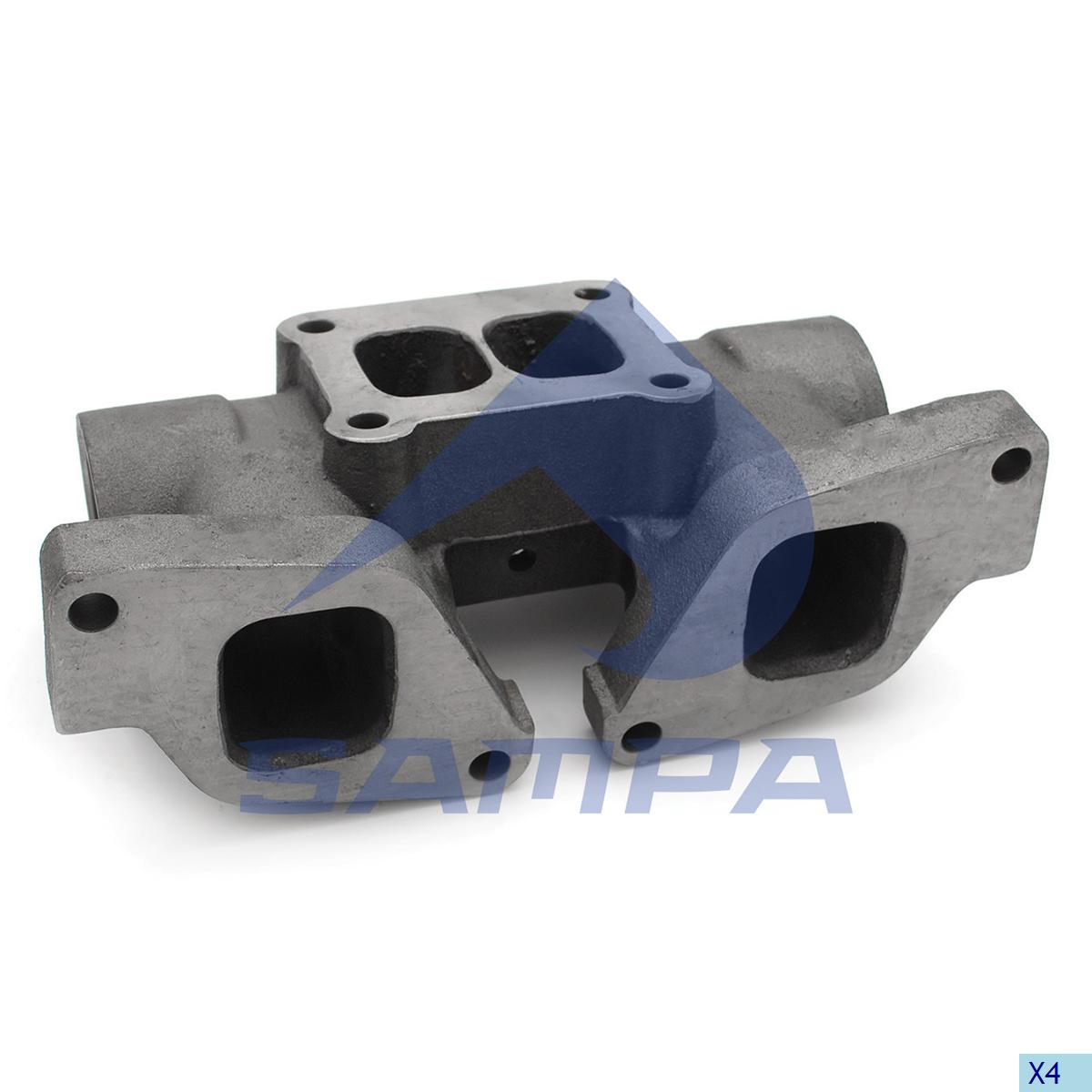The image displays a gray metallic part with a distinct horseshoe-like shape. The part features four square sections, two on the front and two on the top, with circular holes at each corner, potentially for mounting or securing purposes. The interior of these sections appears black, suggesting possible depth or hollow areas within the object. A blue logo with the name 'Sampa' is prominently displayed on the part, with a design pointing to the bottom left of the image. Additionally, there is a blue 'x4' symbol at the lower right corner, indicating a quantity or reference number. The entire scene is set against a white background, creating a stark contrast that highlights the details and design of the object, which could be related to electrical, construction, or automotive applications.